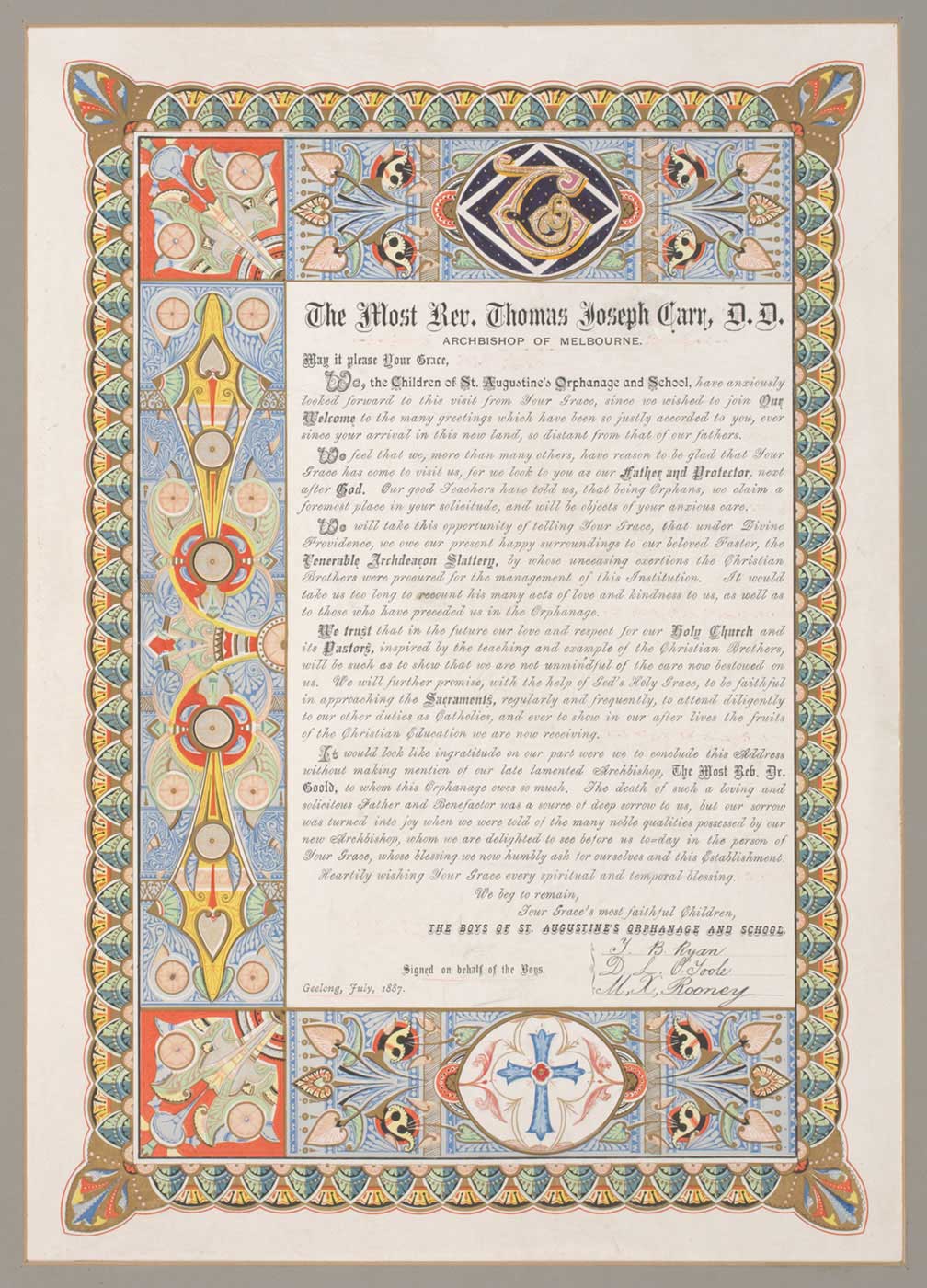The image is of an elaborately designed document that bears a strong resemblance to an illuminated manuscript or a page from the Book of Kells, structured with the formal layout of a diploma. The background consists of a bordered, pastel quilt design in shades of yellow and blue, adorned with intricate floral and geometric patterns. Surrounding the central text are several square panels showcasing a variety of floral and diamond-shaped designs, complemented by a decorative border resembling twisted ropes in hues of blue, green, and yellow with red detailing. 

At the top center of the document, boldly inscribed in black Old English font, is the title "The Most Reverend Thomas Joseph Carr, D.D.," indicating its dedication to an esteemed figure, specifically the Archbishop of Melbourne. The document's rich, decorative framing includes circular motifs, one featuring a notable blue cross with a red center. The detailed scrollwork and decorative elements are executed in pale blue, gold, red, black, yellow, and orange, adding to the historical and intricate quality of the piece.

The main body of the document is filled with tiny cursive print in a calligraphic style, imparting what appears to be a lengthy proclamation or certificate. Signatures are present in the bottom right-hand corner, lending authenticity and a personal touch to the formal document, thus blending elements of both religious and official ceremonial design.